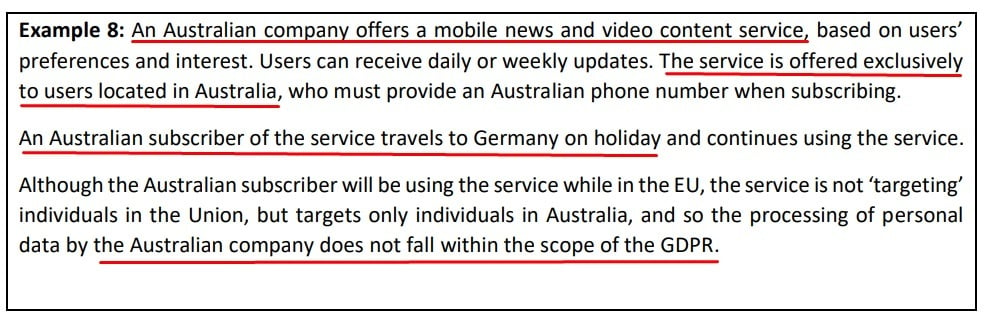**Detailed Caption:**

The screenshot displays a simulation example or a sample question titled "Example 8" in bold black letters located at the top left corner. The text beneath the title describes a scenario involving an Australian company that offers a mobile news and video content service based on users' preferences and interests. It explains that users can opt to receive updates either daily or weekly. The service is available exclusively to users located in Australia, who must provide an Australian phone number during subscription.

The scenario further describes an instance where an Australian subscriber of the service travels to Germany on holiday and continues to use the service. It emphasizes that while the subscriber is using the service within the European Union, the service itself does not target individuals in the EU but is intended solely for individuals in Australia. Consequently, the processing of personal data by the Australian company does not fall within the scope of the General Data Protection Regulation (GDPR).

The background of the screenshot is plain white. Notably, the first sentence, the first sentence of the second paragraph, and the second to last sentence of the first paragraph are underlined in red.